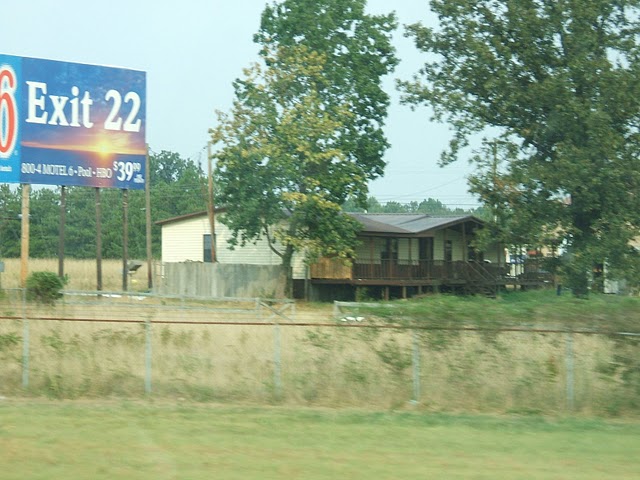A photograph captures a scene of a home situated beside a road. The house, painted in a light beige color, features an architectural design with an arch over the front entrance, followed by another arch in the opposite direction along the length of the building. In contrast to its neutral exterior, the house boasts a dark wooden deck that partially encircles it with a similarly dark wooden fence. The yard surrounding the structure is overgrown with weeds, suggesting a lack of recent maintenance. Just behind the house looms a large billboard that advertises an Exit 22 for a Motel 6, prominently displaying an 800 number—804 Motel 6—and just enough of the sign to reveal the distinctive numeral 6 associated with the motel chain.